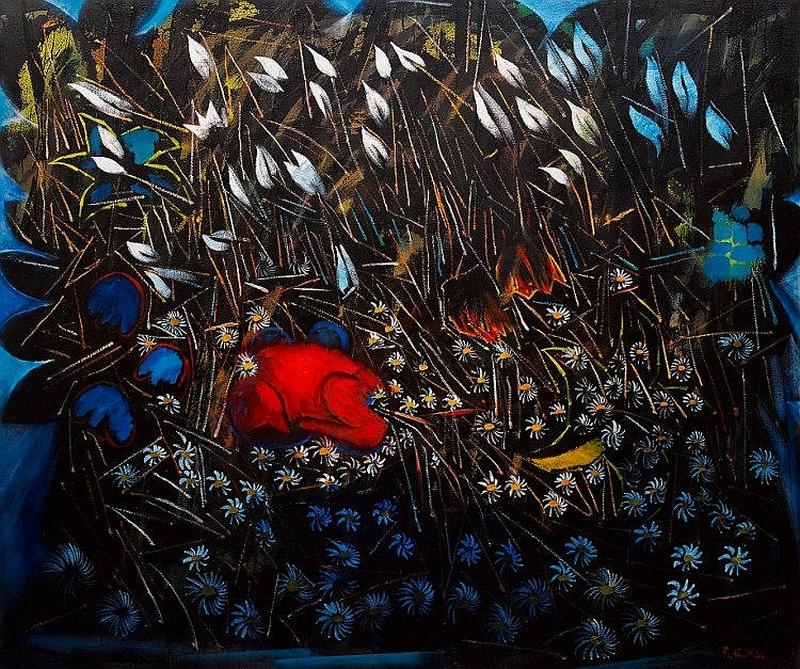This vibrant, striking painting depicts a dark, nighttime scene in a field of tiny daisies with yellow centers and white petals. At the painting's center, contrasting the darkness, lies a bright red animal, possibly a dog or rabbit, curled up in a fetal position among the flowers. The daisies dominate the bottom half of the painting, interspersed with singular white-petaled flowers and blue flowers to the left. Above the flower field, strands of green foliage and spear-like leaves emerge, some standing against what appears to be a rock. In the background, a faint dark blue sky peeks through, suggesting a late evening setting, while the bottom of the painting remains notably darker, gradually lightening as it moves upward.